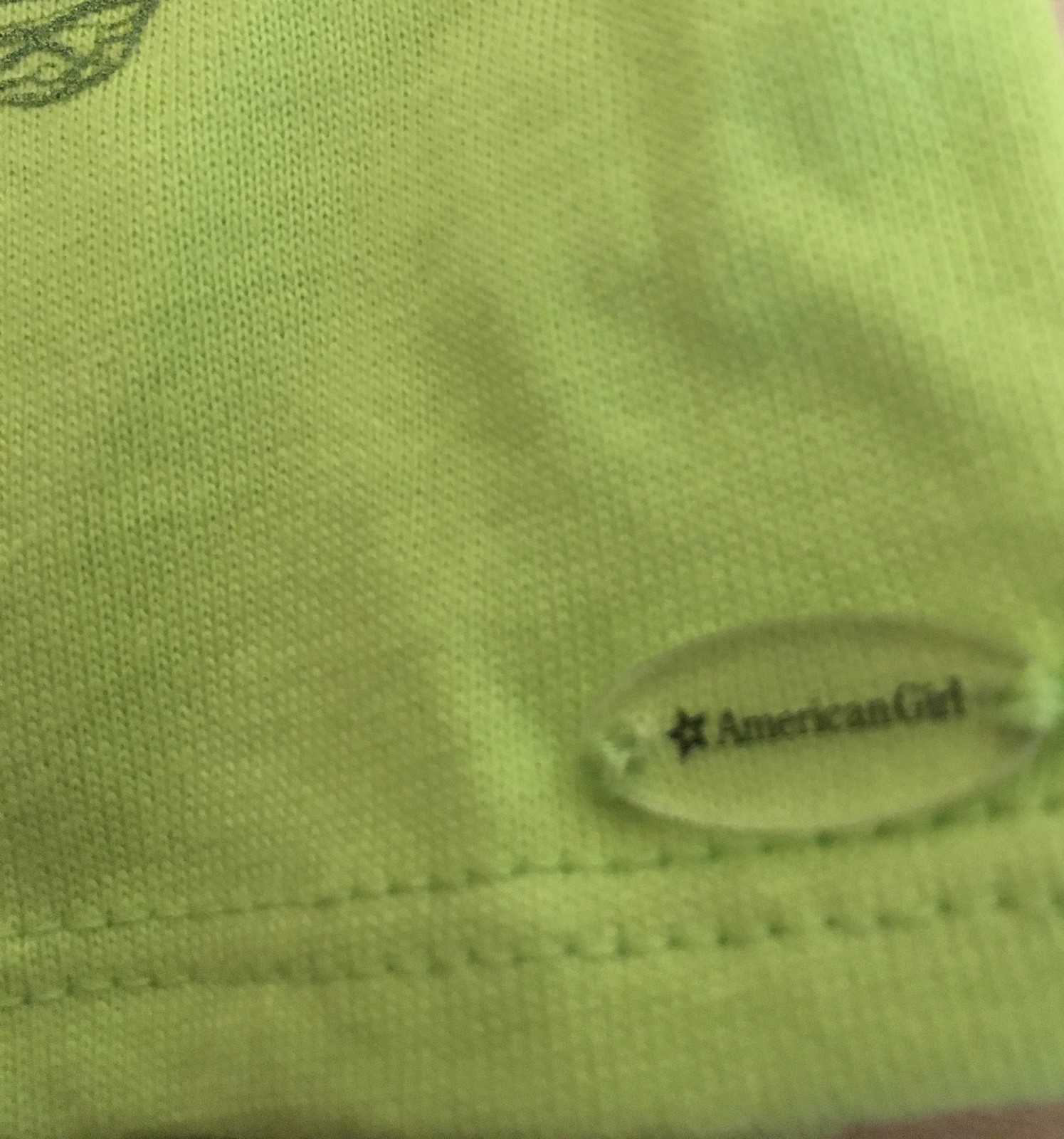The image is a close-up photograph of a small garment, possibly a shirt or blanket, in a vibrant key lime green color. In the bottom right corner of the image, there is an oval-shaped logo positioned sideways, featuring a small black star and the text "American Girl" next to it. Just below this logo, two parallel stitching lines extend horizontally across the fabric. In the top left corner, there is an additional stitched design in dark green. The entire image is zoomed in to highlight this specific section of the garment, showcasing the intricate details and the bright, cheerful color.